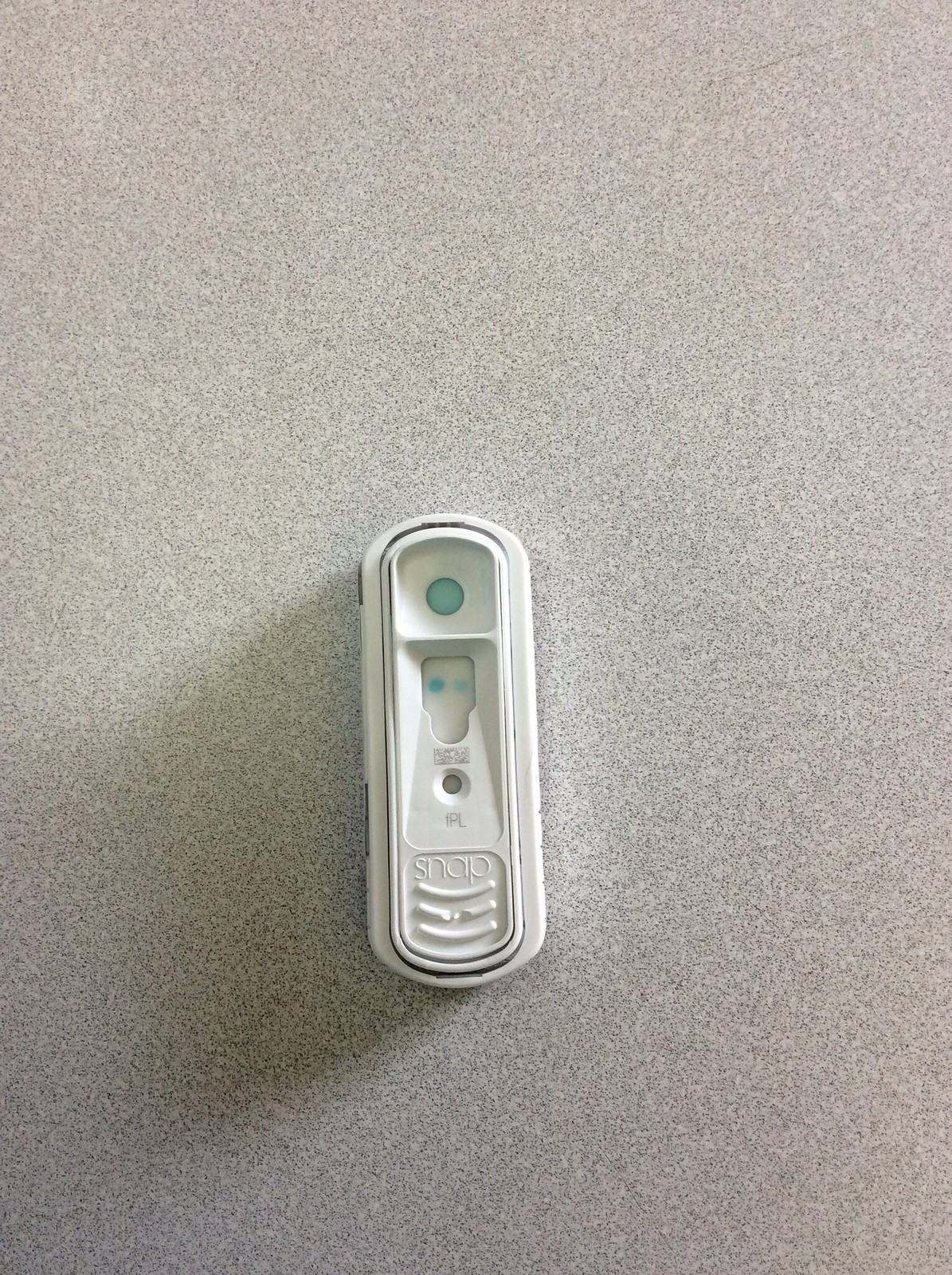The image features a white test device resembling a pregnancy test or possibly a COVID test. At the bottom of the device, the word "Snap" is clearly visible. The design includes several key indicators: a dot at the top, a middle area displaying two light blue dots, and another dot towards the front, which is likely intended for applying a liquid sample. The top dot is entirely filled with a light blue color, indicating an activated test. The two light blue dots in the center suggest a positive result, which typically signifies pregnancy for a pregnancy test or a positive diagnosis for a COVID test. The test is placed on a gray countertop or table, serving as the neutral background for the device.